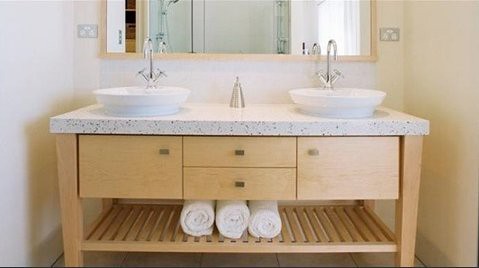This image showcases a traditional his-and-hers sink vanity set in a serene bathroom setting. The base of the unit is crafted from light wood and features an open slatted shelf at the bottom, where three neatly rolled white towels are stored. The countertop is a robust, thick marble surface, providing a sophisticated contrast to the wooden base.

On either side of the countertop are elegant white basins, each accompanied by tall, gracefully arched faucets. The faucets have handles protruding from both the left and right sides at their base, adding to the functional design of the sinks.

Above the sinks is a large mirror reflecting a glass shower door in the background. The door is designed to slide open, with overlapping sections bordered by defined edges, allowing smooth operation from one end to the other. 

Electrical units are visible on both the left and right sides of the mirror, possibly serving as outlets or light switches, though their exact function remains unclear.

The vanity is equipped with cabinet doors and drawers adorned with small, rectangular handles in what appears to be a silver or medium brown hue, contributing a subtle yet stylish detail to the furniture. The surrounding walls are painted in an off-white shade, with areas that appear to take on a beige hue, possibly due to shadowing. This detail enhances the overall warmth and tranquility of the space.